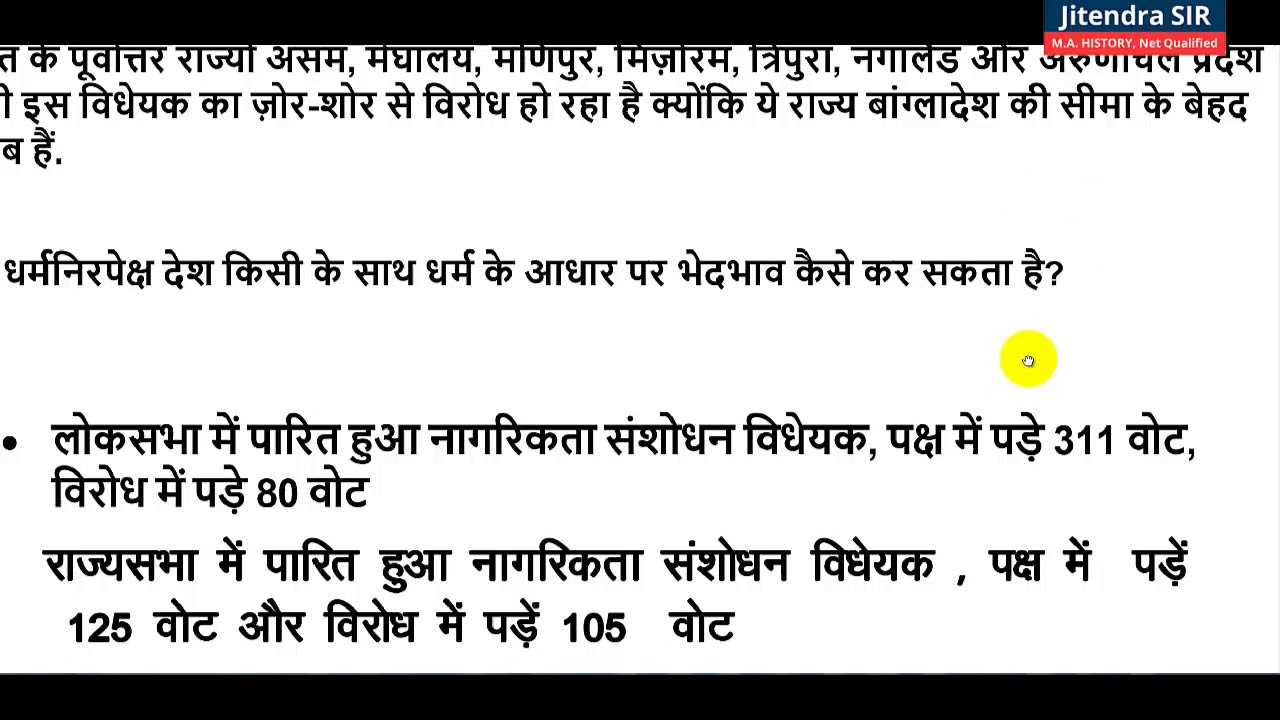A screenshot of a webpage features prominent black horizontal bars at the top and bottom, framing the content. The central section, which occupies a white background, is filled with text in a non-Latin script, possibly Hindi or an Eastern European language. The text is organized into 7-8 lines, with notable spacing between each line at the top and subsequent text below. On the upper right-hand side, the name "Jitendra SIR" is prominently displayed, with "MA History, Net Qualified" written in a red rectangle underneath. The bottom left corner of the image shows the number "125". Additionally, a yellow circle, resembling a mouse indicator, appears near the middle right of the image.